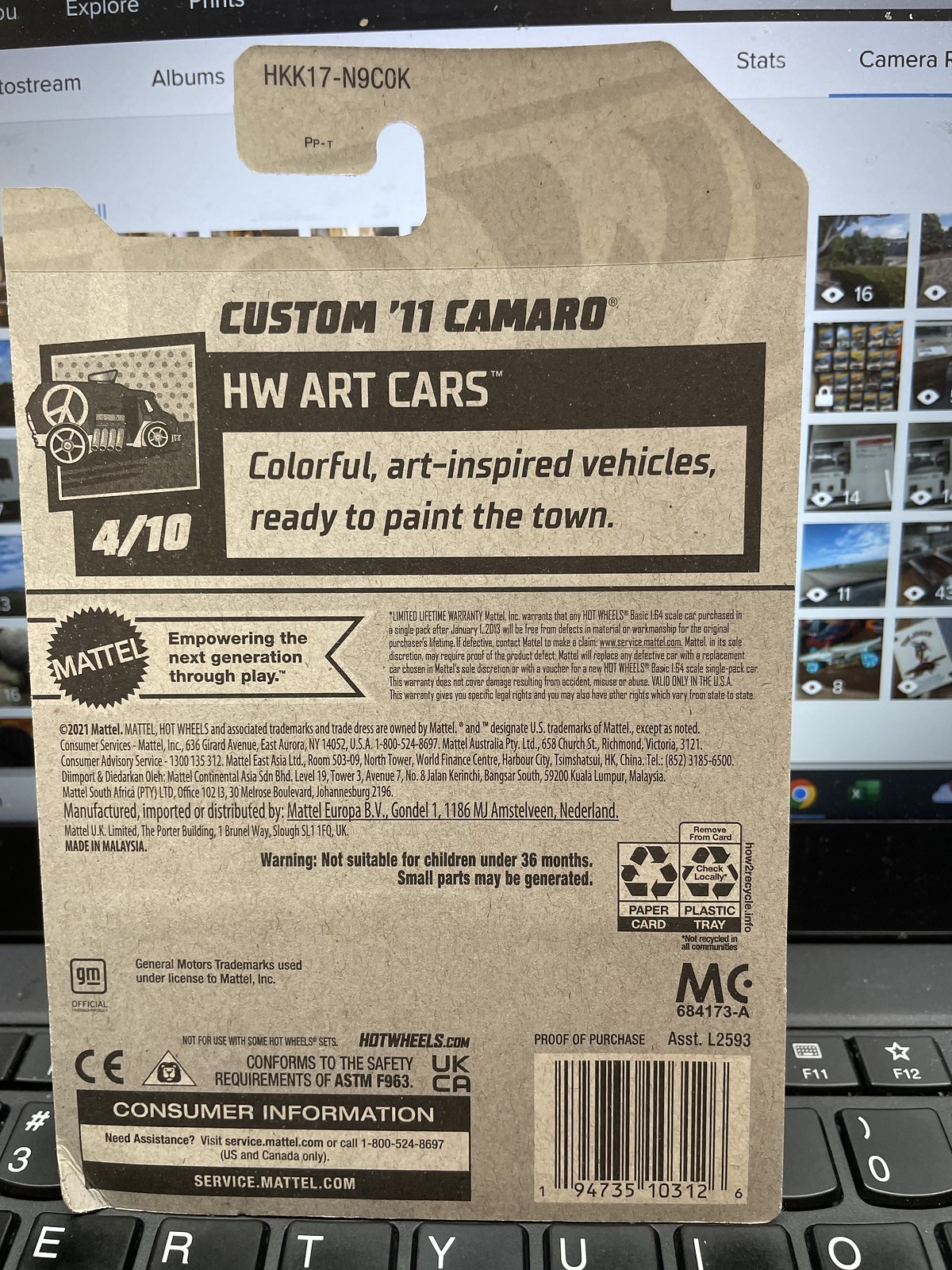This detailed image depicts a placard resting on a keyboard, strategically placed above the E-R-T-Y-U-I-O keys and in front of the number keys, right above the QWERTY section. The placard appears to be designed for hanging, similar to something you'd hang from a windshield or rear-view mirror. It features a rectangular white sticker with black print.

At the top, the sticker prominently reads "Custom '11 Camaro." Directly beneath this, it states "HW Art Cars" against a black background, followed by the text "Colorful art-inspired vehicles ready to paint the town." To the left of this text is a small illustration of a van, which suggests that the product is a toy. Below the image of the van, it is rated 4 out of 10. Underneath this, in a slightly larger font to the left, it reads "Empowering the next generation through play." Centrally placed on the sticker is a spiky circle that includes the Mattel logo.

The lower section of the placard contains a lot of small, unreadable text, which likely includes safety information and product details. A warning label indicates that the toy is not suitable for children under 36 months due to small parts that may be generated, posing a choking hazard. In the bottom right-hand corner, there is a barcode, and to the bottom left, consumer information is listed. The background of the image is a computer keyboard, and at the top right, there are very small, colorful images, less than the size of a postage stamp, depicting various scenes.